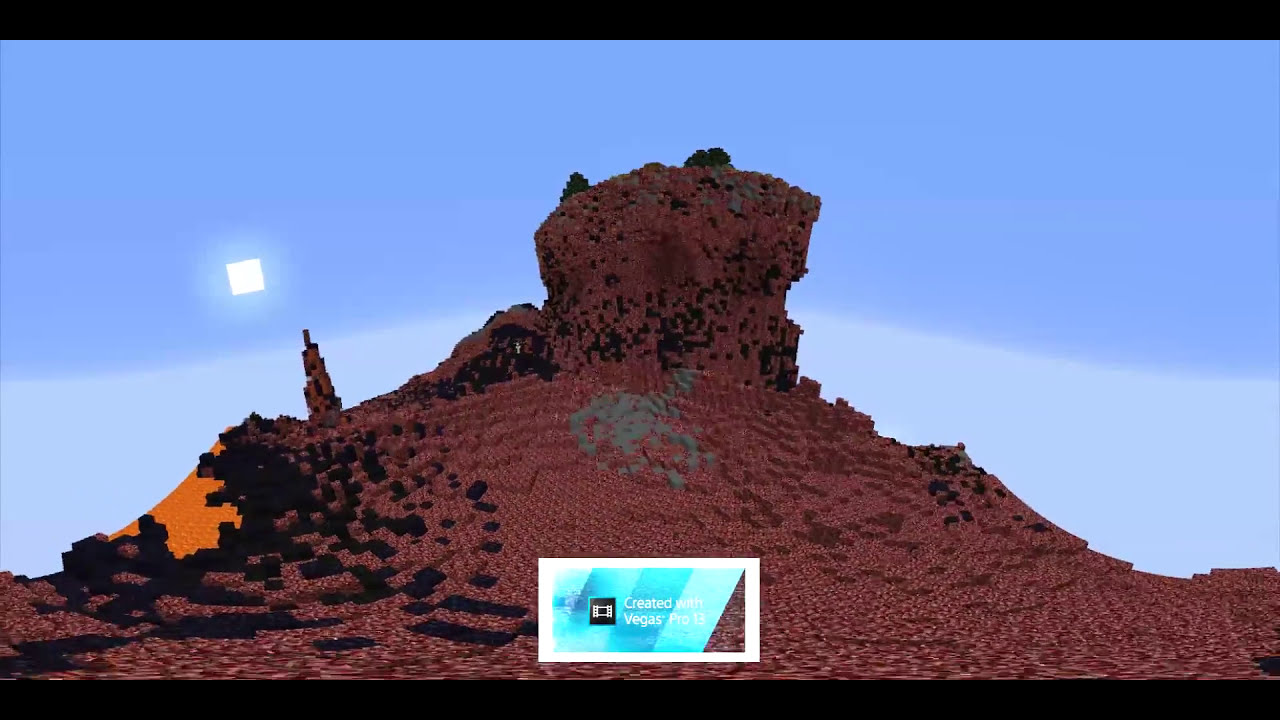The image is a digitally generated, pixelated depiction of a large rock outcropping or rocky hill, characterized by its irregular mound shape and exaggerated pixelation. The hill is mostly composed of bare dirt and rock in various shades of violet, purple, and maroon, with distinguishable patches of black, orange, and gray. A steeper bluff, nearly as high as the hill itself, stands prominently at the center, adorned with a couple of sparse shrubs or trees. The sky behind the hill transitions from pale blue near the horizon to a darker shade higher up, and includes a stylized, white square sun. A noticeable jagged gap on the left side of the hill reveals an orange slope behind. At the bottom of the image, there's a rectangle that reads "Created with Vegas Pro 13," suggesting the use of video editing software. The overall pixelation and framing of the image give the impression of a screenshot from a video game.